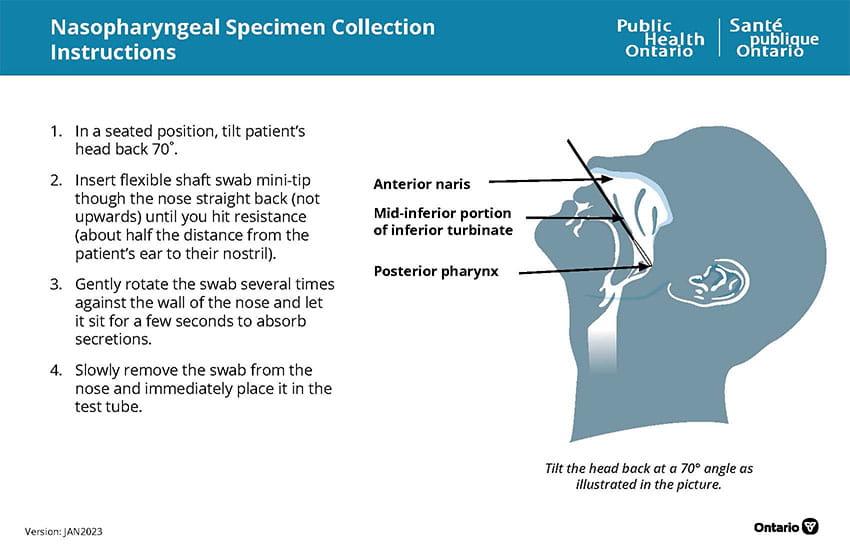The image is a detailed public health informational poster from Public Health Ontario, also labeled in French as Santé Publique Ontario, titled "Nasopharyngeal Specimen Collection Instructions." The poster provides step-by-step guidelines for collecting a nasal specimen. The background is white with a blue title bar and a light blue shaded diagram area. The instructions are as follows: 

1. **In a seated position, tilt the patient's head back 70 degrees.**
   
2. **Insert a flexible shaft swab with a mini-tip through the nose straight back, not upwards, until you encounter resistance, approximately halfway between the patient's ear and nostril.**

3. **Gently rotate the swab several times against the nasal wall and let it sit for a few seconds to absorb secretions.**

4. **Slowly remove the swab and immediately place it in a test tube.**

To the right of these instructions, there is a detailed diagram of a person with their head tilted back, showing the insertion of the swab. The diagram is labeled with anatomical landmarks such as the anterior narus, mid-inferior portion of the inferior turbinate, and posterior pharynx, and it is captioned with "tilt the head back at 90 degree angle, as illustrated in the picture." This visual aid clarifies the correct positioning and pathway for the swab.